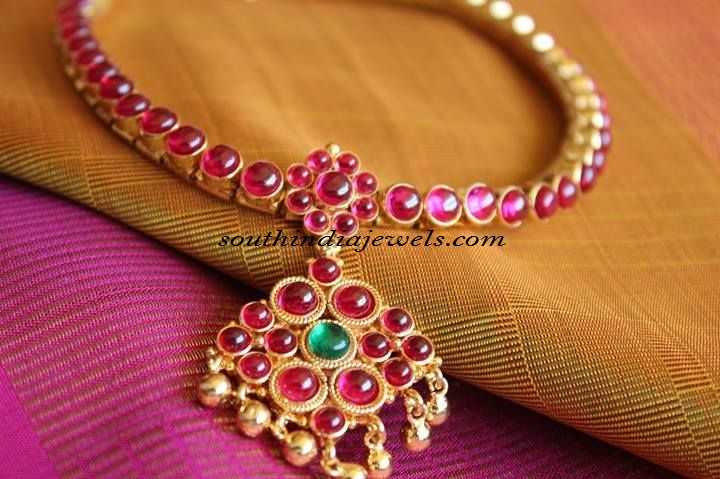This image is a detailed jewelry advertisement showcasing a pink beaded bracelet and a gold necklace, prominently featuring magenta-colored jewels. Set against a vibrant backdrop, the bottom layer consists of bright pink cloth interwoven with golden threads, topped with an orange cloth adorned with darker threads.

The bracelet itself is composed of numerous pink beads interspersed with glass embellishments and features a unique charm. The charm includes a smaller floral design on the bracelet part and a dangling diamond-shaped piece encrusted with pink jewels and a central green jewel. Surrounding the charm are tiny gold balls that add a delicate touch.

In the upper portion of the image, the gold necklace stands out with its magenta-hued, spherical jewels that reveal a green interior. The brand's name, SouthIndianJewels.com, is prominently displayed in black italics with a serif font over the bracelet.

Overall, the image is a rich tapestry of colors and textures that highlights the intricate design of the jewelry pieces against a luxurious fabric backdrop.